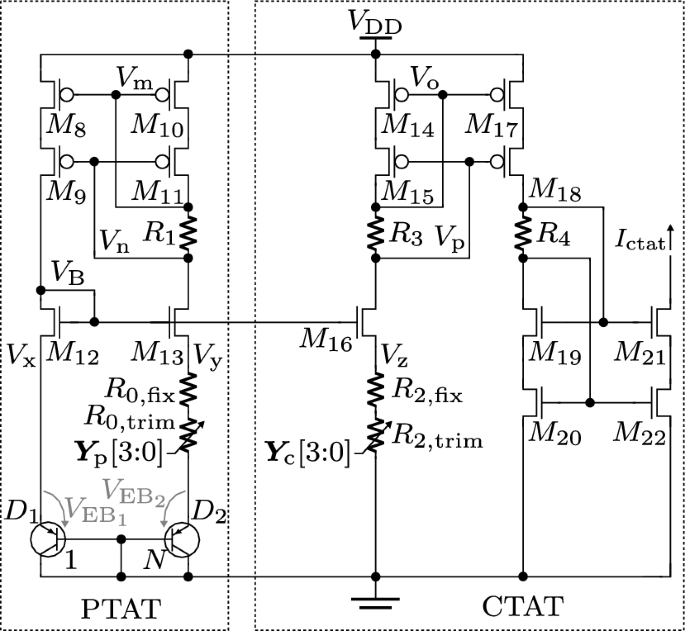This black and white diagram illustrates a 2D electronic circuit on a white background. The circuit consists of various black lines, including solid lines, dotted lines, and lines with circles (both filled and open). There are numerous components such as resistors, switches, and grounding points, each labeled with distinctive identifiers like V_sub_X, M_sub_12, M_sub_13, V_sub_Y, V_sub_B, M_sub_9, R_sub_1, R_sub_2_fix, R_sub_2_trim, R_sub_3, and more. Resistors are marked with "R," and specific labels include PTAT and CTAT at the lower left and right corners respectively. PTAT and CTAT designations correspond to the two main sections of the circuit, with the right section being significantly larger, approximately twice the size of the left section. This detailed schematic is densely packed with technical annotations, ideal for those with specialized knowledge in electronics.